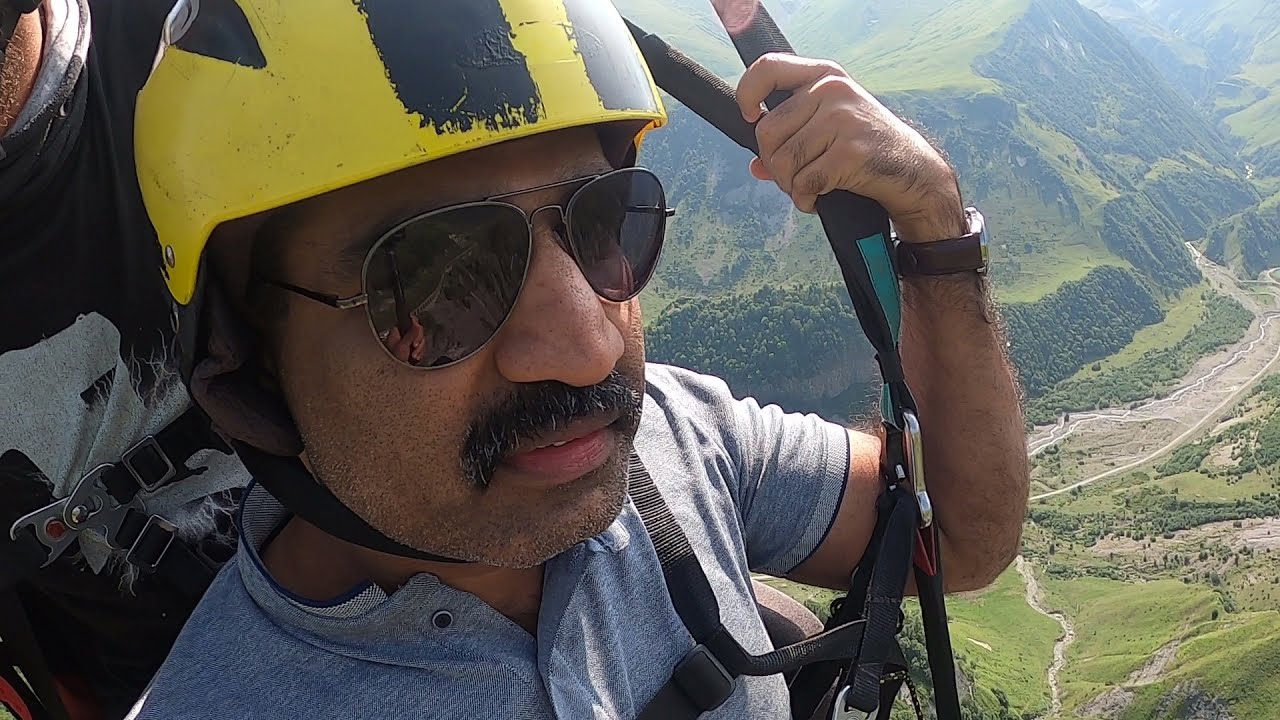The wide rectangular image captures a thrilling moment of skydiving, prominently featuring a man on the left side from his shoulders up, framed against a stunning aerial view of the landscape below and to the right. The man appears to be of Indian descent, with dark hair, a black and gray mustache, and serious expression hidden behind his sunglasses. He wears a distinctive yellow and black helmet, accompanied by a gray shirt and a wristwatch. Secured in a harness, the man grips it with his left hand, indicating the intense push of wind and gravity of the dive. Behind him, another man in a black shirt is just barely visible. The breathtaking background reveals a patchwork of green grass, light beige trails, dark green forests, green hills, and potentially a river, all framing a picturesque mountainous region beneath them.